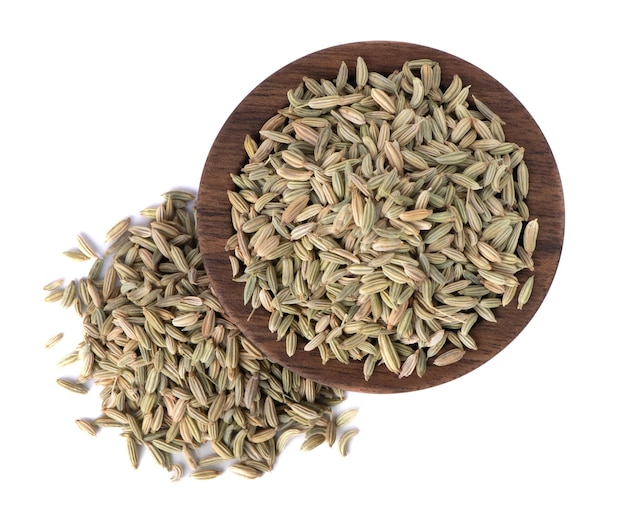This image features a dark mahogany-colored wooden bowl displaying visible wood grains, set against a pristine white background. Inside the bowl, there is a generous amount of long, full kernels that are a mixture of light green and light brown in color, suggesting they might be husked grains or seeds like sunflower or fennel. Additional kernels, in similar hues, are scattered to the left side of the bowl, creating an equal amount of produce both inside and outside the container. The white background, devoid of any text or borders, sharpens the focus on the textured wooden bowl and the vibrant mixture of grains, forming a strikingly minimalist yet richly detailed composition.